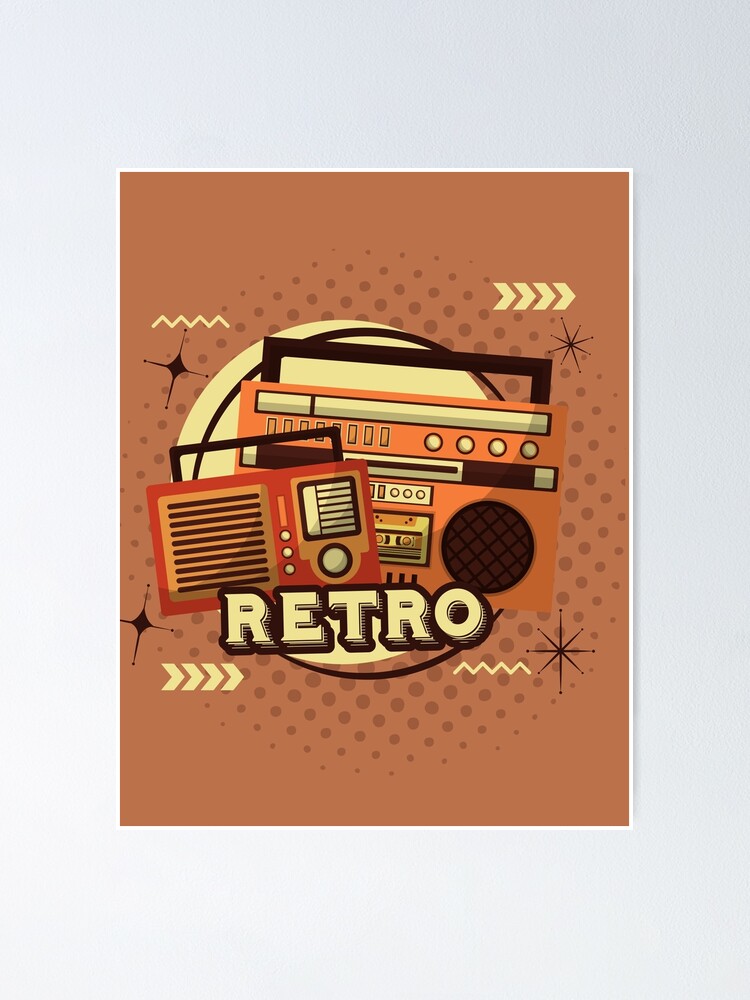The image features a retro-themed stock poster framed by a thick white border. The poster's background is predominantly a rusty brown color with a prominent yellow circle in the center, surrounded by a brown outline. The word "RETRO" is boldly displayed in large, yellowish font outlined in black. Below this text, there are two vintage audio devices: on the left, a smaller red radio with a black handle, characteristic of the 50s or 60s, featuring a turn button and speaker; on the right, a larger boombox with orange and brown detailing, including white knobs and a cassette window. The design is accentuated with abstract patterns, including yellow polka dots, arrows, and squiggly lines, giving the poster a vibrant, nostalgic feel reminiscent of older styles of listening to music. The entire composition sits against a very light lavender background, adding to its retro charm.